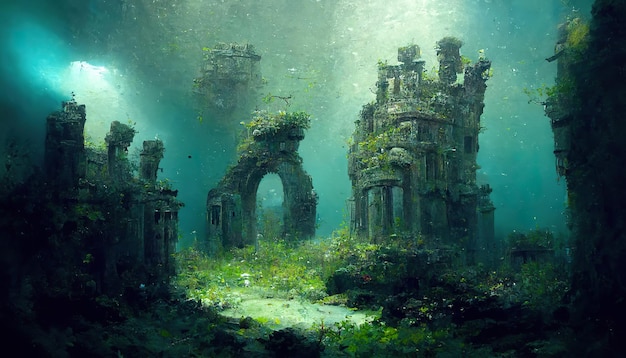This image is an underwater scene captured in a detailed, watercolor painting. At the forefront lies an ancient, submerged village, with structures on both the left and right sides. The focal point is a prominent archway slightly to the left, possibly leading to a garden or porch area. To the right stands what seems to be a temple, approximately a story and a half tall, crafted from rough, gray stone. The remnants of old homes and other buildings give the impression of a once-thriving settlement, now reclaimed by the sea. 

Marine growths, including grass and moss, abundantly cover the stone ruins, indicating they have been underwater for quite some time. The water has a grayish-green hue, filled with floating debris, creating an authentic underwater ambiance. Sunlight filters down from above, illuminating select areas and casting a serene glow on the green spaces between the structures. The ground is carpeted with aquatic plants, enhancing the scene's lushness. Despite the absence of sea creatures, the painting's impressionist style breathes life into the ancient, medieval-like ruins, evoking a sense of quiet beauty and timelessness.